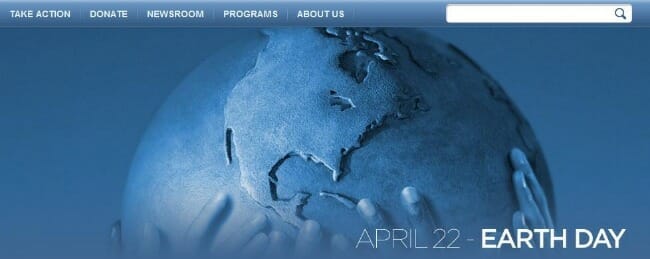This image is a screenshot or photograph of a website, predominantly featuring varying shades of blue. Central to the image is a partial depiction of the globe, rendered in blue with illuminated accents, suggesting a glowing effect. Beneath the globe, several blue hands, some overlapping and numbering three or four, are shown reaching upwards as if to grasp the globe, symbolizing unity and collective effort.

In the bottom right corner, the image prominently displays the date "April 22nd" in white letters, and just above this, in bold white typography, the words "Earth Day" are clearly visible, signifying the theme of the depicted event. Near the top of the image, a navigation menu is present, listed in white bold letters, including clickable links labeled "Take Action," "Donate," "Newsroom," "Programs," and "About Us," all clearly standing out against the background.

Additionally, the top right corner features a search box outlined in white, accompanied by a magnifying glass icon, indicating an interactive feature for conducting searches. The lighting of the image suggests a source emanating from the bottom left, casting a gradient that lightens this area while gradually darkening towards the top right, enhancing the visual depth and focus on the globe.

Overall, the image evokes a sense of global awareness and collective action pertaining to Earth Day, supported by clear visual cues and purposeful design elements.